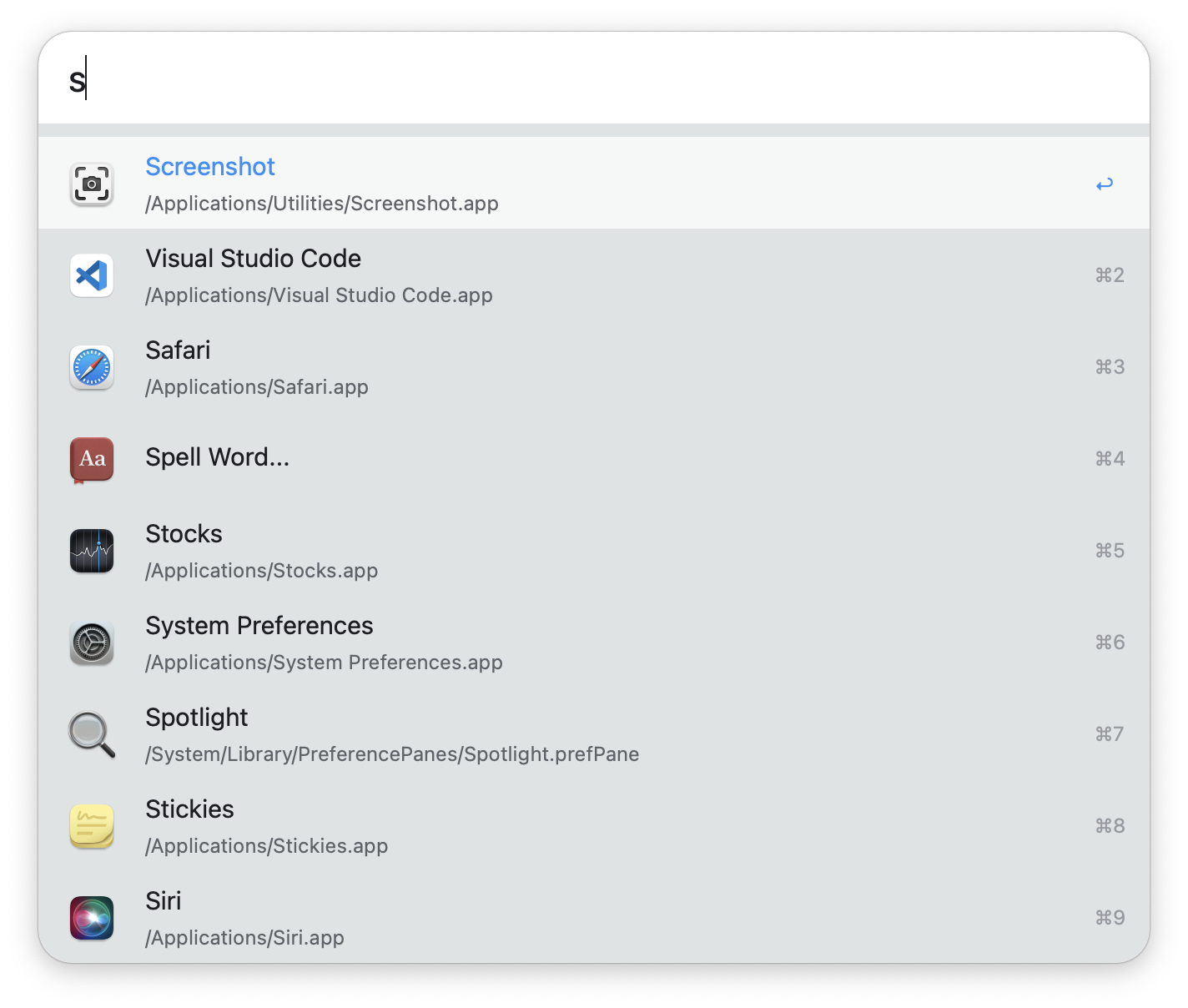The image features a grayscale interface with various application details. At the top, there's a white box with a bold black "S" followed by a line. Below it, a light gray, illuminated box reads "Screenshot" accompanied by a small application icon. Directly next to this is a blue left-pointing arrow.

The darker gray section presents a list of applications, each followed by their respective file paths and frequency markers:

1. **Visual Studio Code**: Displayed with an "X" and the number "2," indicating "applications/visualstudiocode.app."
2. **Safari**: Listed alongside "applications/safari.app" with a "×3."
3. **Spell Word**: Denoted by "×4."
4. **Stocks**: Mentioned with the path "applications/stocks.app" and marked "×5."
5. **System Preferences**: Found under "applications/systempreferences.app" with a "×6."
6. **Spotlight**: Detailed as "system library preference panes/spotlight.prefpane" with a "×7."
7. **Stickies**: Noted with "applications/stickies.app" and a "×8."
8. **Siri**: Listed as "applications/siri.app" with a "×9."

These elements are methodically aligned and coded to signify their respective applications and usage instances, set against the minimalistic gray backdrop.